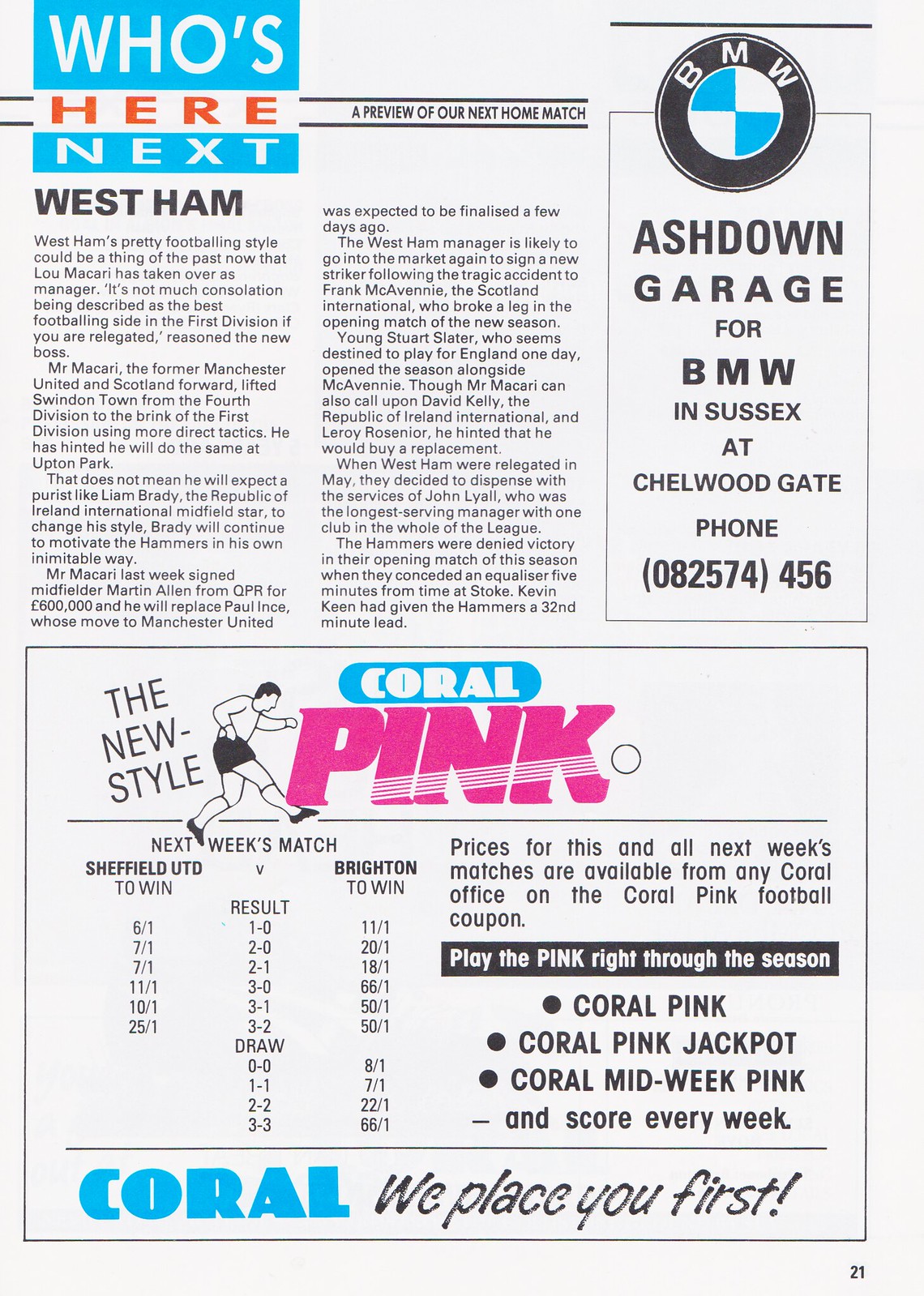This image appears to be a page from a soccer magazine or program, designed in a vertical rectangular format. The top section features a segmented title reading "Who's Here Next" with "Who’s" in white on a light blue background, "Here" in red on a white background, and "Next" again in white on a light blue background. Directly below this title, the page announces the upcoming team, West Ham, in bold black letters.

To the right of this title, the BMW logo is prominently displayed, and beneath it, an advertisement for Ashdown Garage for BMW in Sussex, which includes the location (Chelwood Gate) and phone number (082-7574-46).

The main body of the page consists of two columns filled with text providing a detailed preview of West Ham's next home match, including their schedule and familiar facts about the team. The lower half of the page transitions into marketing content for Coral Pink, described with a variety of colors and typography. The text indicates an upcoming match between Sheffield United and Brighton, recent match results, and details about Coral Pink’s offerings, hinting that it may be a gambling or betting service closely associated with the soccer matches.

Additionally, the page features illustrations and logos interspersed within the content. The Coral Pink advertisement section includes a drawing of a soccer player kicking a ball, with Coral’s slogan, "the new style," and further promotional phrases emphasizing their betting services, such as "Coral Pink Jackpot," "Coral Midweek Pink," and admonitions to "play the pink right through the season."

In summary, the detailed and visually dynamic page mixes game previews, advertising, and promotional content, prominently featuring West Ham, BMW, and Coral Pink, and is likely part of a soccer program or magazine designed for match attendees.